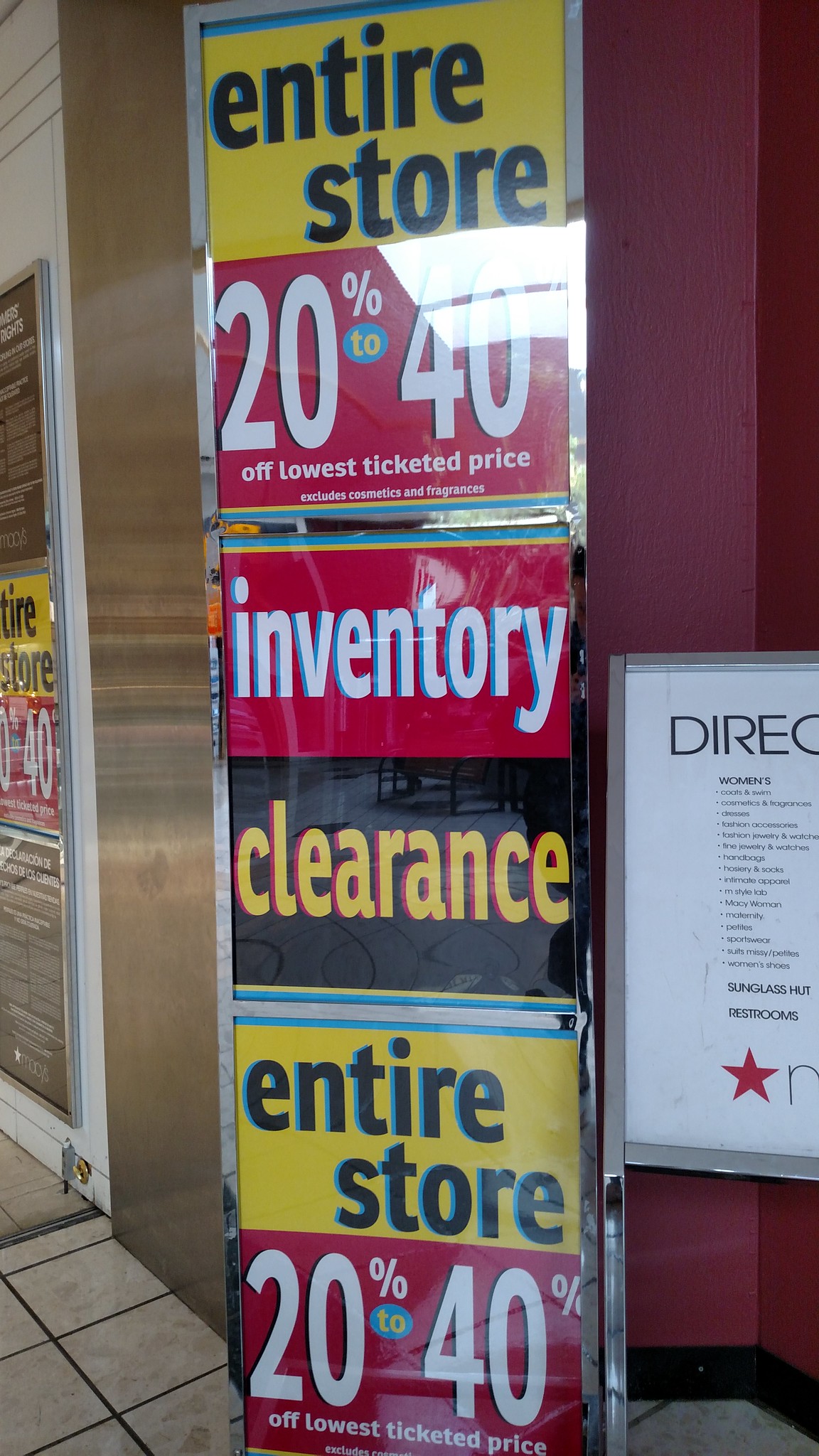The image depicts a tall sign stand located near the entrance or exit of a Macy's store. The stand has a sleek, silver, chrome-like border that gives it a modern look. The sign inside announces an "Entire Store 20-40% Off" sale, emphasizing "Off Lowest Ticket Price" and "Inventory Clearance." The text is vibrant, using a mix of yellow, red, and black colors to grab attention. To the right of this stand, there is another sign, enhancing the promotional display. The backdrop is a burgundy-colored wall, adding a sophisticated touch to the scene. The store's floor features neatly arranged, white, square tiles, completing the clean and orderly presentation.